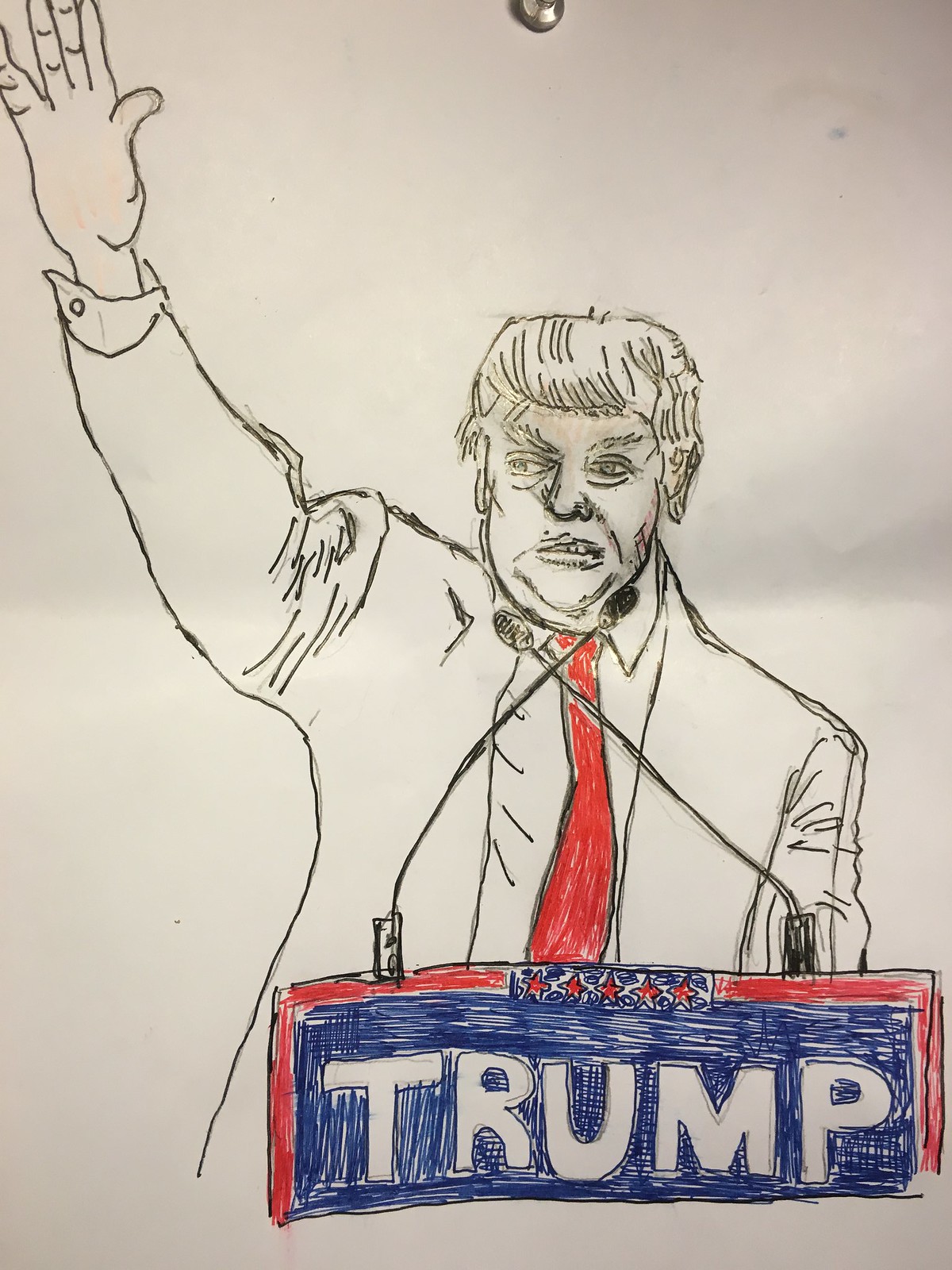This image is a vertically oriented drawing of Donald Trump, likely during a campaign. The illustration appears to be hand-drawn on a white sheet of paper, which seems to have been crinkled and possibly folded. At the very top center of the paper, there is an object resembling a magnet.

Trump is depicted standing at a podium, facing the viewer, with his right hand raised in the upper left-hand side of the drawing. His gaze is directed off to the left. He is dressed in a jacket over a shirt, and he sports a red tie. His left hand rests below the podium.

Two microphones, crossing each other like an "X", are positioned near his mouth. The podium itself is outlined with a red border, followed by a blue box. Inside this blue box, "TRUMP" is written in white letters. Above the podium, five red stars are arranged within the blue box, adding a patriotic touch to the scene.